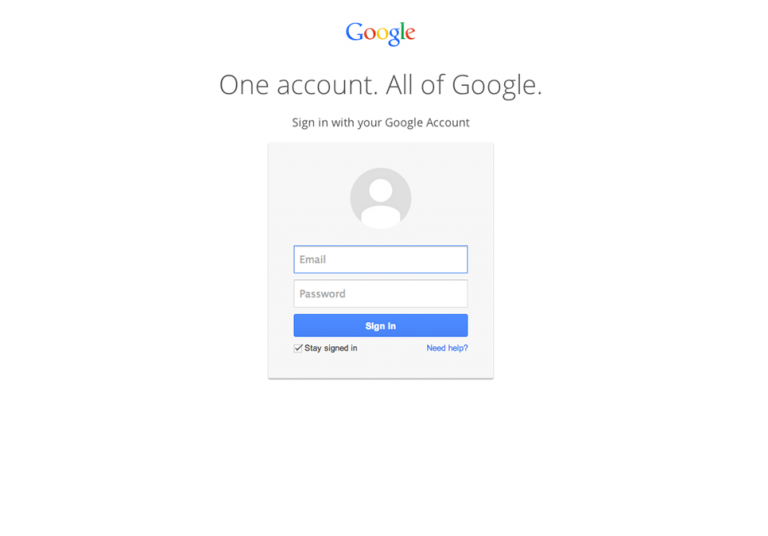Screenshot of Google Sign-In Page

The image displays a Google sign-in page with a clean, white background. At the top of the page, the recognizable Google logo appears in a mix of blue, red, yellow, and green colors. Below the logo, gray text reads "One account. All of Google."

The main content of the page features a light gray box, which includes a gray circle icon resembling a person. Directly beneath this icon, there's a rectangular field labeled "Email" for users to input their email addresses. Below the email field is another rectangular box labeled "Password" for password entry.

Towards the bottom, there's a blue rectangular button with white text reading "Sign In." Beneath this button, there's an option with a check box labeled "Stay signed in." Additionally, a blue link at the bottom reads "Need help?"

The layout is minimalistic, intended to facilitate straightforward user interaction for signing into a Google account.